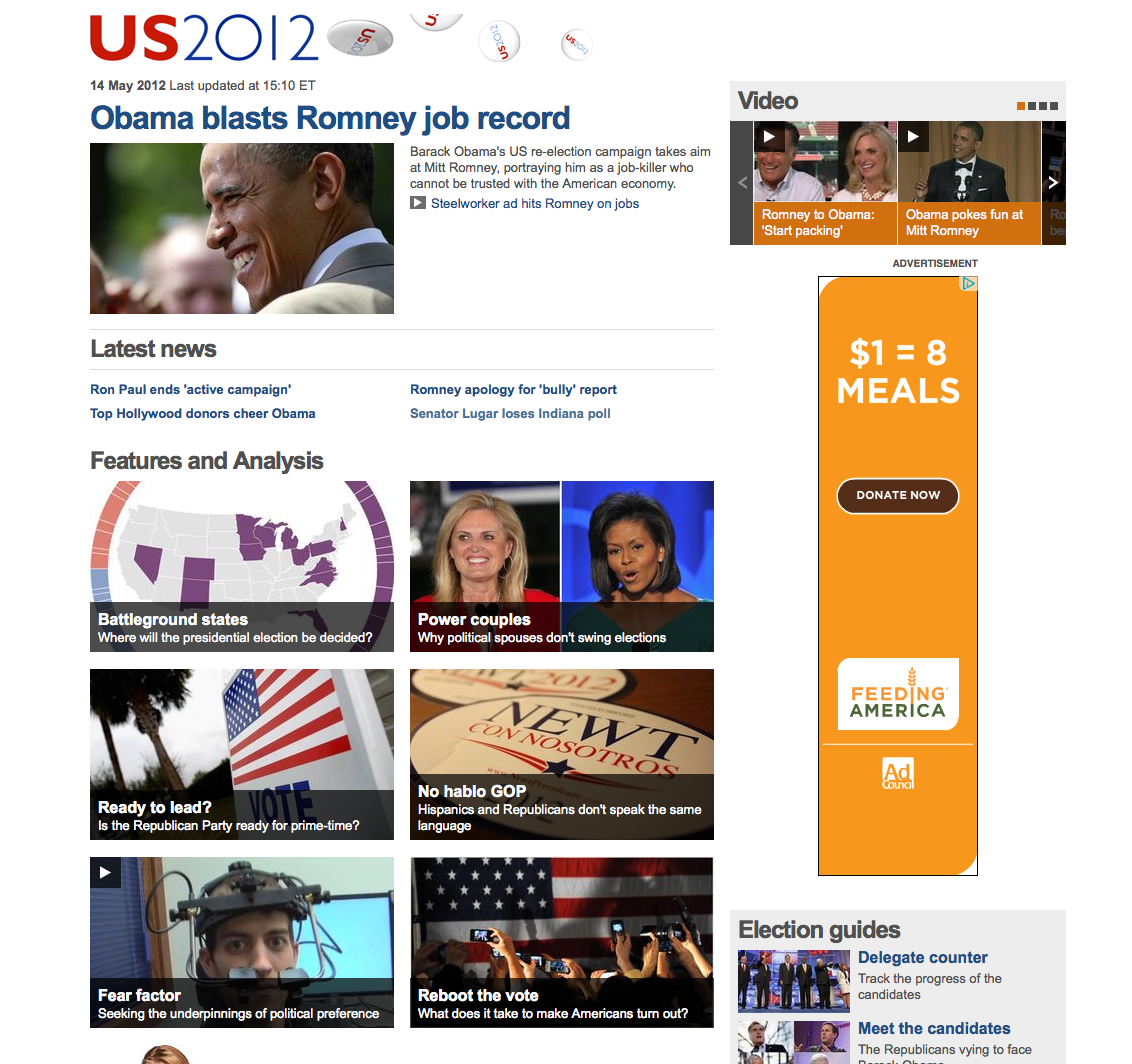The image captures a snapshot of a news webpage from May 14, 2012, which was last updated at 3:10 PM. At the top of the page, the headline reads "U.S. 2012" with a subheading that highlights "Obama blasts Romney's job record." Below this headline is a photo of Barack Obama. 

Adjacent to the image of Obama is a video thumbnail featuring Mitt Romney and his wife. Next to this video is another picture captioned "Obama pokes fun at Mitt Romney," indicating that there is a video available to watch on the website.

Further down the page under "Latest News," the following headlines are visible:
- "Ron Paul ends active campaign"
- "Top Hollywood donors cheer Obama"
- "Romney apology for bully report"
- "Senator Lugar loses Indiana poll"

At the bottom, the "Features and Analysis" section presents various topics:
- "Battleground states: Where will the presidential election be decided?" 
- "Power couples: Why political spouses don't swing elections," accompanied by a photo of Mitt Romney’s wife and Michelle Obama.